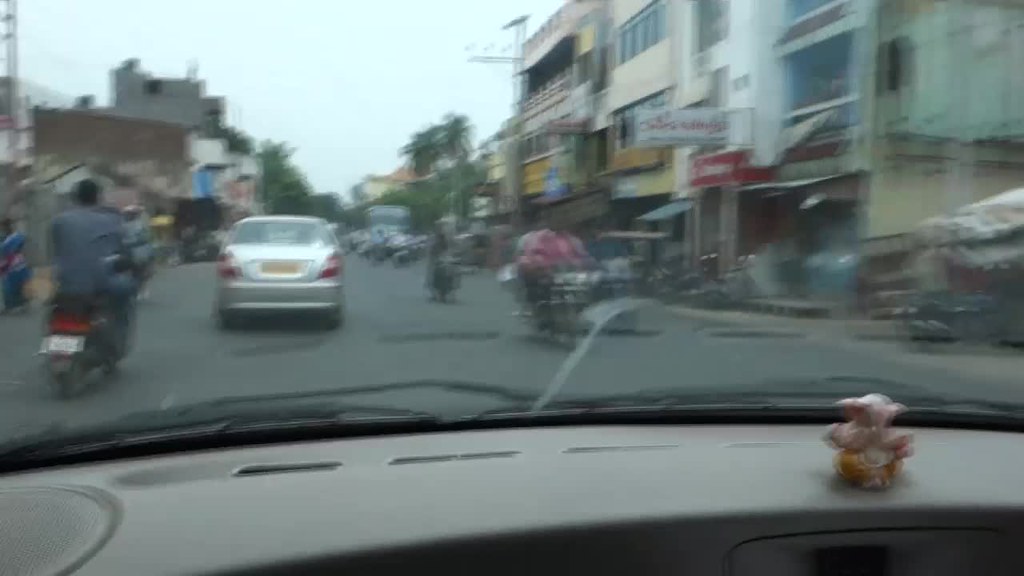This photograph, taken from inside a car through the windshield, captures a bustling street scene in a foreign city during the daytime. The street is dominated by an array of motorcycles and mopeds outnumbering the few cars present, including a prominent silver car with a yellow license plate. The cityscape is framed by tall, green trees interspersed between buildings on both sides of the street, which appear to be storefronts, adorned with various signs. The vividness and height of the trees add a splash of greenery to the urban environment. The car's dashboard and windshield wipers are faintly visible in the foreground. Above it all, the light blue sky with patches of overcast adds to the atmospheric depth, slightly blurred in the distance, which enhances the sense of motion and daily life in the photograph.